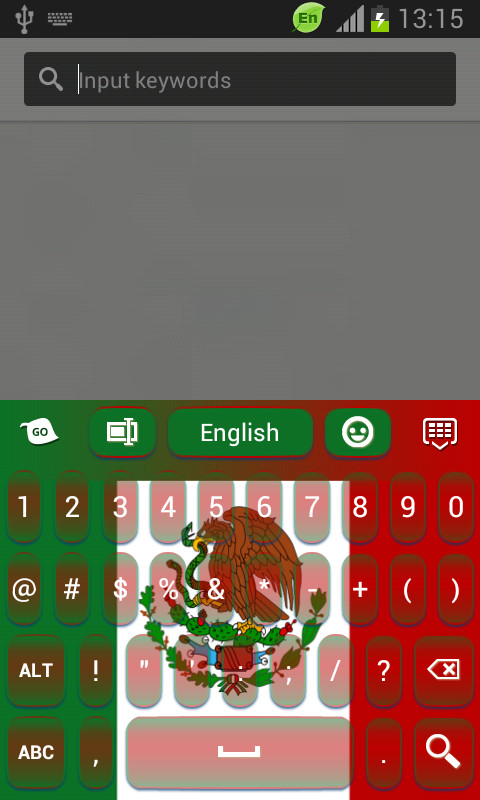The image depicts an early keyboard with a unique and colorful design. The keyboard fades from green on the left to red on the right, giving it a vibrant appearance. Overlaid on this color gradient is an illustrated, cartoon-like representation of a brown falcon, which is facing sideways and appears to be eating a green worm.

The top part of the keyboard has a grayscale color scheme, transitioning to the colorful gradient below. The interface displays various elements, including a gold leaf symbol and a rectangle with a cursor hovering over it. The selected keyboard format is English. Other visible elements include an emoji, a calculator, and the standard set of keys, with numbers on the front row.

At the very top of the image, there's a status bar displaying important information such as the battery life, which is denoted by a green leaf, and the current time in military format, showing 13:15. Below that, the input area for keywords is delineated. It features a black box where input text appears in gray.

The unique combination of elements and colors, along with the cartoony bird motif, gives the keyboard a distinctive and playful aesthetic.